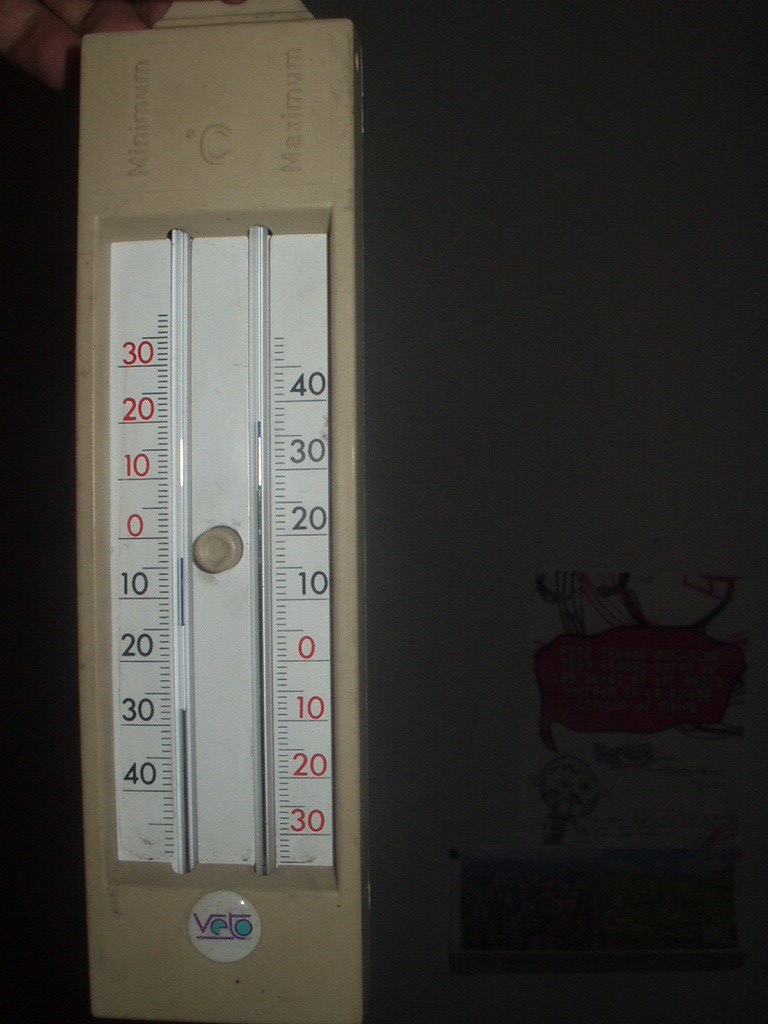The image features an outdoor thermometer encased in a beige plastic rectangular frame. The frame is adorned with various descriptive details and measurements. At the top, the words "Minimum" and "Maximum" are clearly raised from the plastic, along with a degree symbol followed by the letter "C" for Celsius.

The bottom part of the thermometer showcases a circular white area, prominently displaying the brand name "VETO" in purple letters. The interiors of the letters "E" and "O" are filled with turquoise color, adding a distinct touch. 

The thermometer incorporates two measuring gauges. The left gauge is marked with numbers ranging from 30 to 0 in descending order in red print, followed by 10 to 40 in ascending order in black print. The right gauge features numbers from 40 to 10 in descending order in black print, followed by 0 to 30 in ascending order in red print.

Centrally placed between the two gauges, there is a gray or beige push button, presumably for resetting or calibrating the thermometer. The overall design is functional yet detailed, providing precise temperature readings for outdoor monitoring.